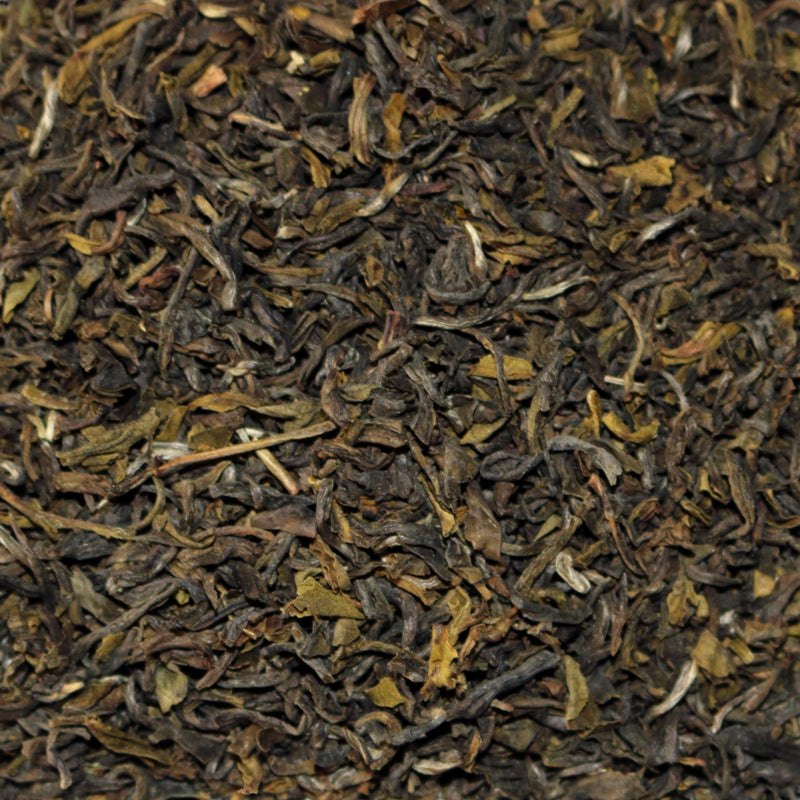The image is a close-up, square-shaped photo capturing an outdoor, natural ground surface that is densely covered with detritus from trees. The scene is dominated by a mix of various shades of brown and yellow, with interspersed hues of tan, gray, white, and nearly black. The ground itself is not visible as it is completely covered by what appears to be a combination of rotting leaves, small sticks, and possibly composted material. The pieces of detritus differ in size and shape, including some that are long and twig-like, others that are curved or straight, and many that resemble dried leaves. The elements are scattered irregularly throughout the image, creating a chaotic, intertwined pattern with no clear order. The overall impression is one of natural decay, with hundreds, if not thousands, of these elements densely packed together, suggesting a forest floor or a wooded yard strewn with debris. The background color appears predominantly dark gray, adding depth to the intricate and organic clutter of the surface.